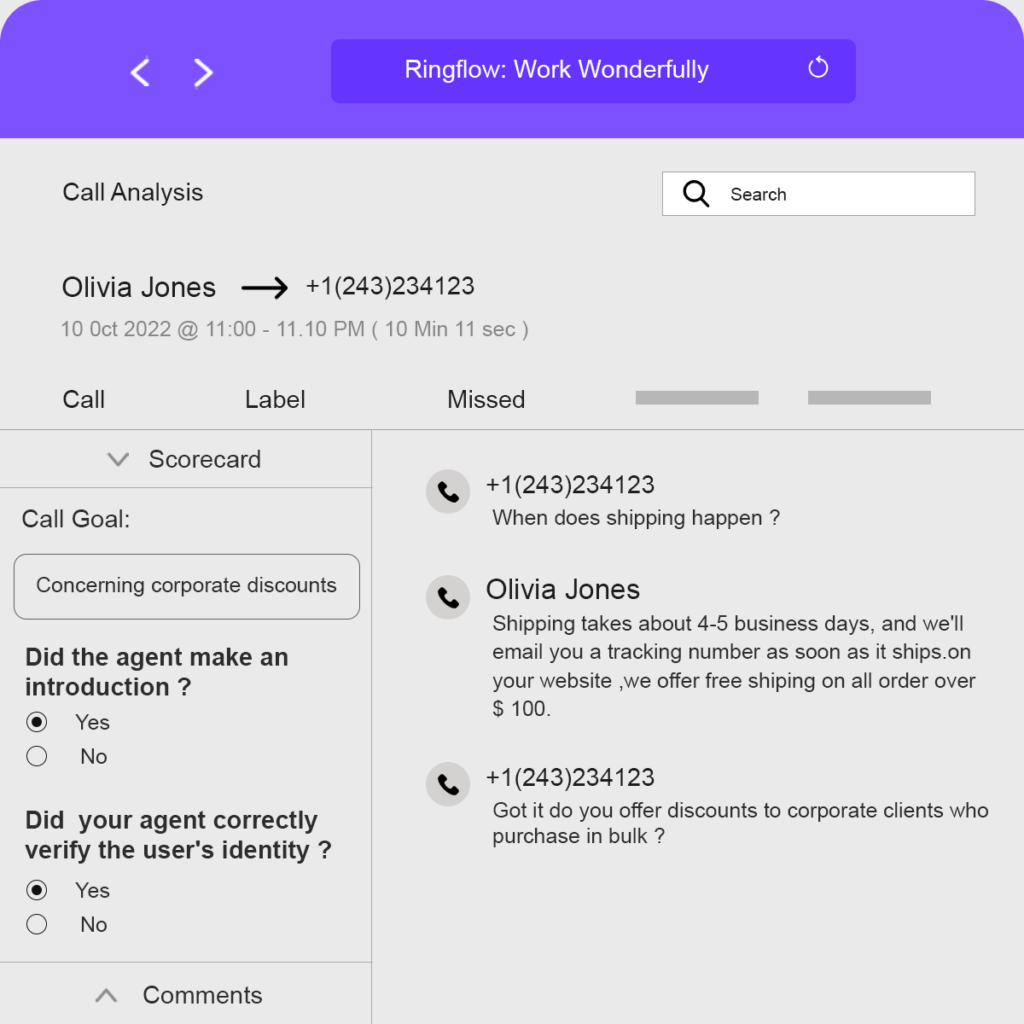**Caption:**

This screenshot showcases a call analysis page featuring multiple sections and interface elements. At the very top is a deep purple bar with a back arrow and a forward arrow on the left side. Just below this, a purple box prominently displays the message "Ring Flow work wonderfully." 

Moving down, there is a gray section headed with "Call Analysis" positioned on the top left. Adjacent to it on the right is a white search bar. Under the heading, the name "Olivia Jones" is displayed with a right arrow leading to the phone number "+1 243-234-1234." Below this, the date appears in light gray font.

Further down, a "Call Label" section is in mist-colored text, followed by a dividing line. On the left side under this line, there's a "Scorecard" section. This includes details such as the "Call Goal" focusing on "Corporate Discounts," and assessment criteria like "Did the agent make an introduction?" with options for 'Yes' or 'No', and "Did the agent correctly verify the user's identity?" also with 'Yes' or 'No' options.